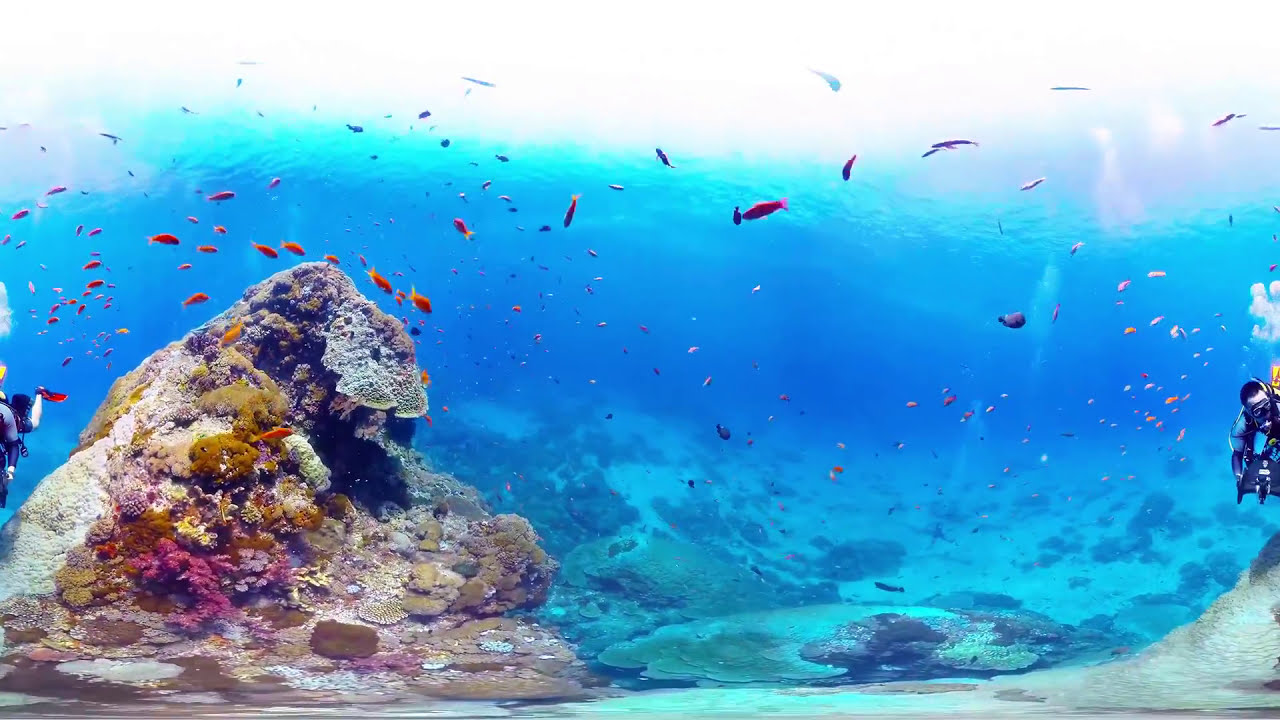This underwater photograph captures a vibrant coral reef scene on the seafloor. On the left side of the image, a large outcropping of corals and various undersea plants, including anemones, showcases a spectrum of colors from neutral grays and blues to golds, pinks, reds, and purples. The coral formations display diverse textures, emphasizing the richness of marine life. Surrounding this outcropping are rocks that appear predominantly blue, their natural hues slightly distorted by the ocean's blue tint. In the distance, dozens of small fish can be seen swimming; they range in color from orange to pink, purple, and blue, and vary in size. The water's color transitions from a dark blue in the background, suggesting great depth, to a lighter blue near the top where the ocean surface is visible. Additionally, two scuba divers are partially visible: one on the extreme left, showing only part of their head and breathing apparatus, and another on the far right, where you can see part of their face, dark black hair, and blue diving shirt. The scene is a mesmerizing display of underwater life, enriched by the interplay of light and color.